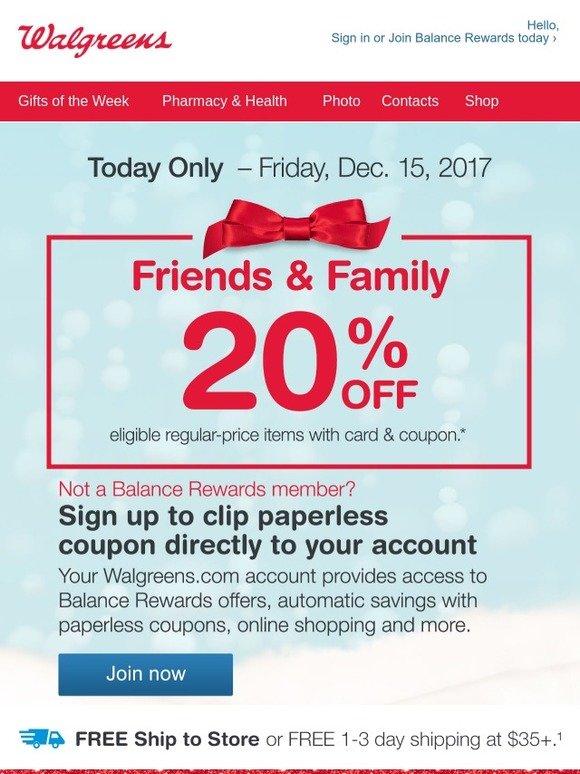The image is a screenshot taken from a computer displaying a promotional banner for Walgreens. At the top, "Walgreens" is prominently written in a decorative cursive font in red. To the right, there is a message in blue inviting customers to "Hello, sign in or join Balance® Rewards today."

A red banner with tabs runs across the top of the image, featuring options labeled "Gifts of the Week," "Pharmacy & Health," "Photo," "Contacts," and "Shop." The background of the banner is blue with a visual effect of falling snowflakes, creating a festive holiday atmosphere.

The banner designates "Today Only" in bold black text, specifying the date as "Friday, December 15th, 2017." Below this text, a visual of a satin ribbon tied in a bow encircles a red box. Inside the box, it reads "Friends and Family 20% off eligible regular price with card and coupon."

A red text statement highlights "Not a Balance® Rewards member?" followed by black text explaining the benefits of signing up: customers can "clip paperless coupons directly to your account," gain access to "Balance Rewards offers," enjoy "automatic savings with paperless coupons," and facilitate "online shopping and more."

At the bottom of the promotional content, there is a blue "Join Now" button for viewers to click and enroll in the rewards program.